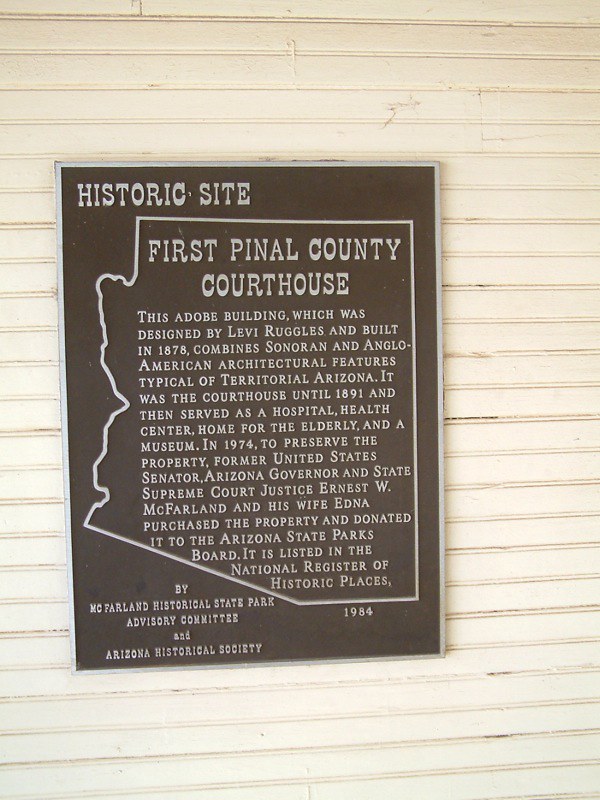This image shows a plaque attached to a wall composed of horizontal wooden planks painted in a soft white color, resembling shiplap or siding. The metal plaque, which has a brown background and a silver frame, features a white sketch outline of the state of Arizona. Above this outline, the text reads "Historic Site," while inside the state shape, it states "First Pinal County Courthouse." The sign provides detailed historical information, explaining that this adobe building, designed by Levi Ruggles and built in 1878, combines Sonoran and Anglo-American architectural features typical of Territorial Arizona. It served as the courthouse until 1891 and subsequently functioned as a hospital, health center, home for the elderly, and a museum. In 1974, Ernest W. McFarland—a former United States Senator, Arizona Governor, and State Supreme Court Justice—along with his wife Edna, purchased the property to preserve it and donated it to the Arizona State Parks Board. The site was listed in the National Register of Historic Places in 1984, as noted by the McFarland Historical State Park Advisory Committee and the Arizona Historical Society.